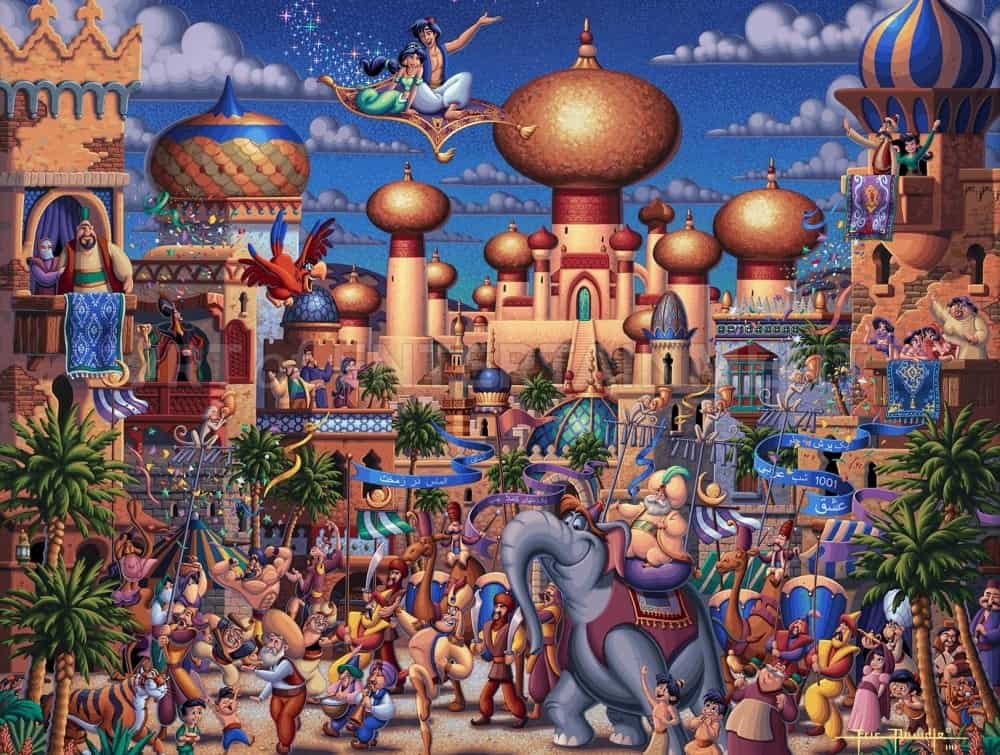This horizontal, richly detailed image appears to be a handmade or digitally animated scene inspired by the Disney franchise of Aladdin. At the top, Aladdin, dressed in a blue jacket and white pants, and Jasmine, clad in a light green outfit, soar through the bright blue sky on their iconic magic carpet, amidst fluffy white clouds. Below them sprawls the ornate kingdom of Agrabah, characterized by its distinctive beige buildings with bulbous tops and intricate metalwork, evocative of a scene from the animated Aladdin movie of the 1990s.

The bustling cityscape is teeming with life as if a grand festival or parade is unfolding. The ground and rooftops are crowded with nearly a hundred vibrant figures, including notable characters, animals, and townsfolk dressed in period-appropriate attire. Prominent among them is the Sultan, wearing flowing beige robes, riding a grey elephant adorned with a red vest and a tuft of red hair. This chaotic yet festive atmosphere includes a tiger, children, and other exotic creatures like camels, all adding to the scene's rich tapestry of colors and activities. The backdrop features a grand palace with multiple towers and balconies where people wave to the crowd below, enhancing the sense of a celebratory spectacle. Notably, the genie is absent from this scene. The image encapsulates the lively essence of Agrabah, depicting Aladdin showing Jasmine the world from their unique vantage point high above the joyous crowd.